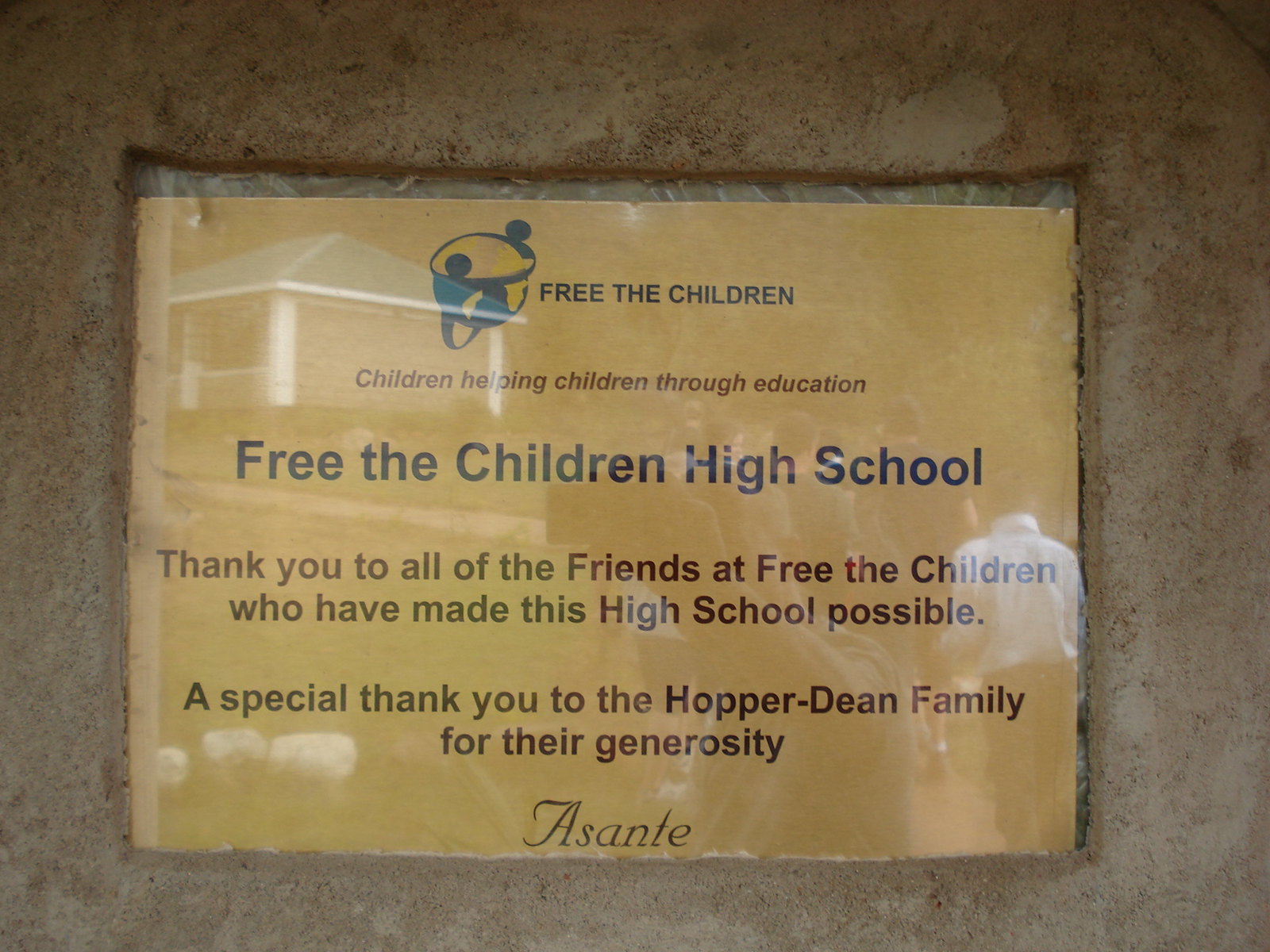The photograph captures a rectangular tribute plaque encapsulated in a clear plastic cover, set against a dark brown stone or stucco background. The plaque is laid out in a landscape orientation and printed on yellow parchment-like paper. At the top, there's a Free the Children logo featuring two children holding hands around a globe. Next to the logo, the text reads "Free the Children." Below this, in lighter print, is the phrase "Children Helping Children Through Education." Prominently displayed beneath this in bold, dark text is "Free the Children High School." Further down, text reads, “Thank you to all of the friends at Free the Children who have made this high school possible. A special thank you to the Hopper-Dean family for their generosity.” At the bottom, centered, the word "Asante" appears in an elegant script. The background of the yellow paper faintly shows an overlay image of children walking up to a school building, although it is subtle and hard to discern clearly. Reflections are visible on the clear plastic cover, adding a layer of visual complexity to the image.